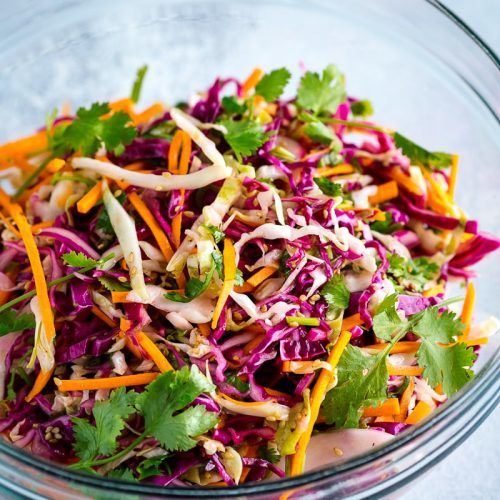A realistic image captures a glass bowl of salad placed on a light blue table. The medium-sized bowl is halfway filled with a vibrant mix of thinly shredded vegetables, predominantly red cabbage, along with a fair share of shredded carrots, and green cabbage. The colorful medley includes scattered pieces of cilantro, also known as coriander, adding green flecks among the purple, orange, and white hues. The cilantro leaves appear to have stems and are roughly torn, not finely chopped, giving a rustic feel to the salad, which resembles a slaw. Though there are hints of yellow seeds sprinkled throughout, the salad does not appear to have any obvious seasoning or dressing, maintaining a fresh and simple look.